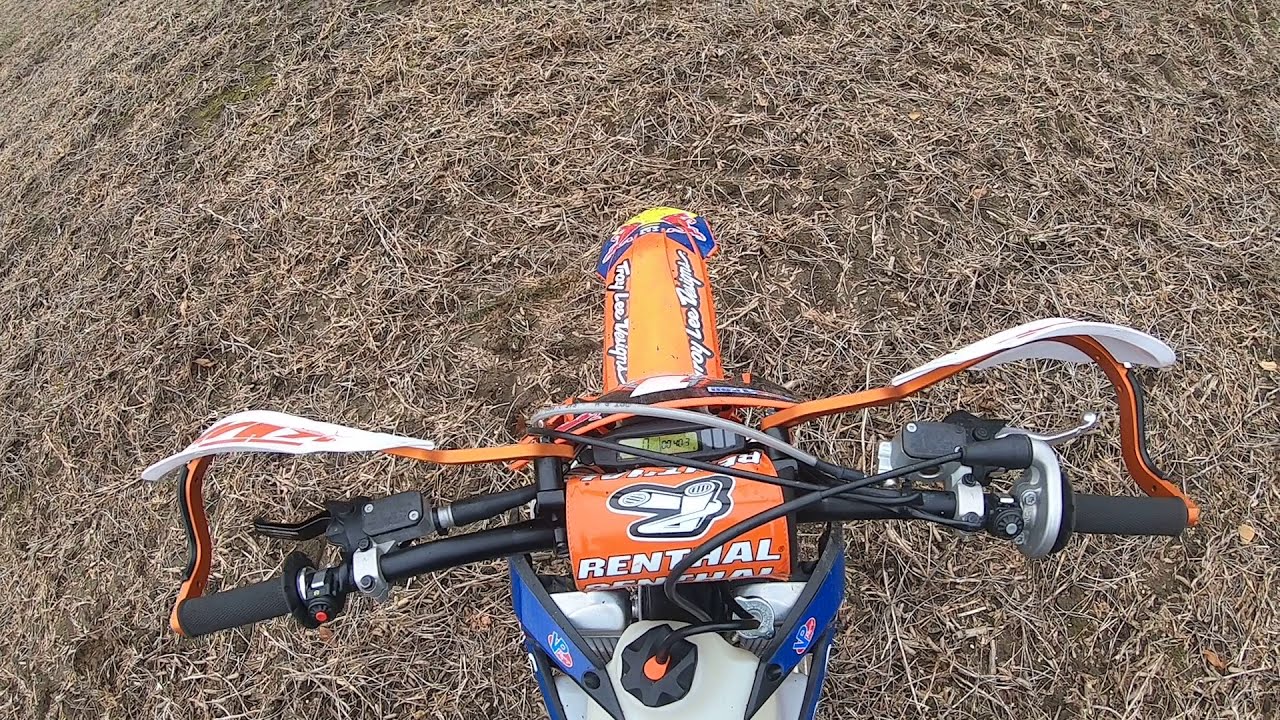This photograph captures the rider's perspective from a dirt bike as they overlook its vibrant, detailed features. Dominating the center of the image is the bike, specifically its orange front fender with blue trim. The handlebars, prominently colored in orange and brandishing the white "Renthal" logo, draw immediate attention due to their central positioning and distinctive branding. Each handlebar is equipped with white and orange hand guards, enhancing both the bike’s functionality and aesthetic. The tank, situated directly beneath the handlebars, showcases a sleek white body with a contrasting black cap, accentuating the bike's overall blue and orange color scheme. Spread out before the bike, the ground is a flat and expansive field, riddled with tire treads and blanketed in sun-dried hay or dead grass, adding a rugged texture to the scene. The dead grass's hues of brown and gray reinforce the outdoor setting's raw, uncultivated character. Additionally, black cables snake their way visibly around the bike's front, hinting at its intricate mechanical structure. In essence, the image vividly illustrates the thrill and ruggedness of the dirt bike riding experience through meticulous attention to both the bike’s detailed components and its surrounding environment.